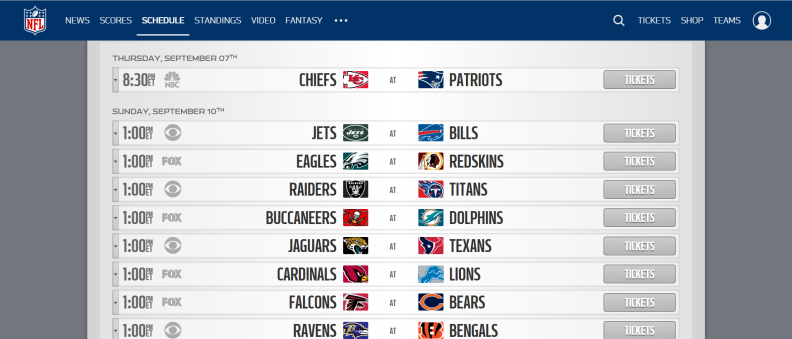A detailed screenshot of the NFL website showcases the official NFL logo prominently in the upper left-hand corner. A well-organized menu bar runs across the top of the page, offering navigation options for "News," "Scores," "Schedule," "Standings," "Video," and "Fantasy." On the upper-right side of the screen, additional options are available for "Tickets," "Shop," and "Teams." Dominating the center of the screenshot is the NFL schedule, which lists upcoming games for different teams. Key matchups include: 

- **Thursday, September 7th at 8:30 p.m. ET:** Kansas City Chiefs vs. New England Patriots 
- **Sunday, September 10th at 1:00 p.m. ET on CBS:** New York Jets vs. Buffalo Bills 
- **Sunday, September 10th at 1:00 p.m. ET on FOX:** Philadelphia Eagles vs. Washington Redskins 
- **Sunday, September 10th at 1:00 p.m. ET on CBS:** Oakland Raiders vs. Tennessee Titans 
- **Sunday, September 10th at 1:00 p.m. ET on FOX:** Tampa Bay Buccaneers vs. Miami Dolphins 
- **Sunday, September 10th at 1:00 p.m. ET on CBS:** Jacksonville Jaguars vs. Houston Texans 
- **Sunday, September 10th at 1:00 p.m. ET on FOX:** Arizona Cardinals vs. Detroit Lions 
- **Sunday, September 10th at 1:00 p.m. ET on FOX:** Atlanta Falcons vs. Chicago Bears 
- **Sunday, September 10th at 1:00 p.m. ET on CBS:** Baltimore Ravens vs. Cincinnati Bengals

All mentioned times are in Eastern Time.